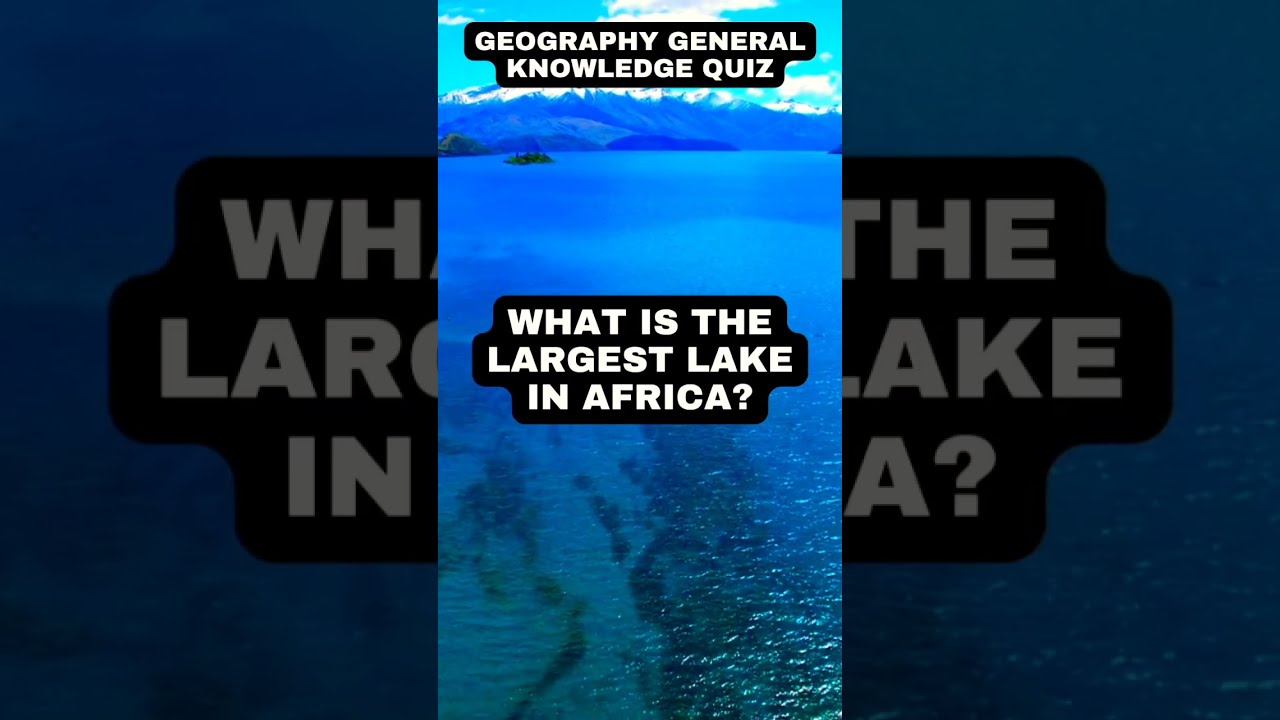The image features a beautiful wilderness landscape divided into three panels. The central panel displays a stunning photorealistic scene of crystal-clear, very blue waters extending into the distance, with numerous dark shapes visible beneath the surface close to the camera. Looking out across the water, a range of snow-capped, dark blue mountains dominates the horizon. The sky above is bright blue, dotted with several white clouds. The right and left panels show zoomed-in and darkened versions of the central image, highlighting details from the sides. In the top third of the central panel, over a small black shape, the words "Geography General Knowledge Quiz" are written in white. Below, in the center of the image over another black shape, the question "WHAT IS THE LARGEST LAKE IN AFRICA?" is prominently displayed in white capital letters. Additionally, there appears to be a small island with vegetation in the water, adding to the scenic beauty of the landscape.